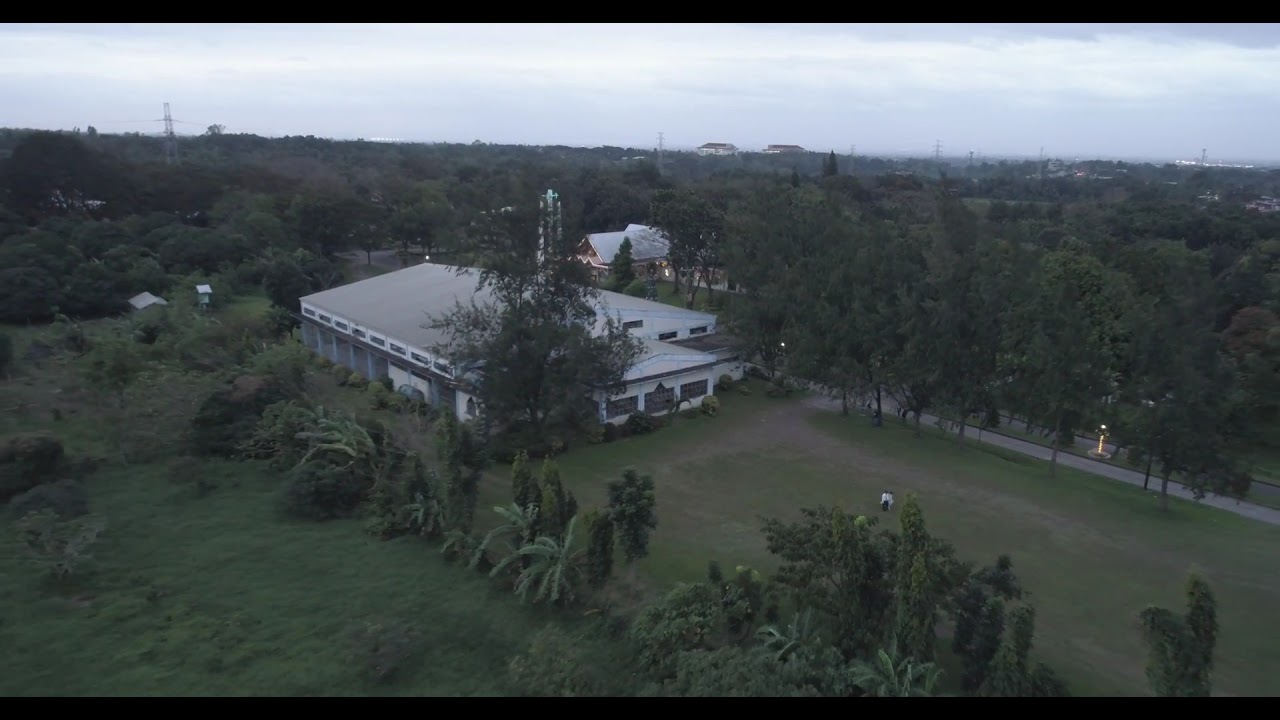A large, white building, possibly a warehouse or a church, dominates the image from a drone's overhead perspective. The structure features a flat, gray roof with white accents and large rectangular windows along its sides. A tall tree grows close to the building, partially obscuring a sign beneath it. There is a two-story building with its lights on situated behind it, hinting at dusk as the blue sky begins to darken. Surrounding the main building, there is lush greenery with a mix of smaller decorative trees and tall, tropical-like trees. The area is heavily wooded, with additional buildings scattered among the trees and a prominent tower on the left. Power lines can be sporadically seen in the distance. A road and sidewalk parallel the building, extending from the right side of the image. Overall, the photo captures a blend of natural and man-made elements in a semi-rural setting transitioning into the evening.